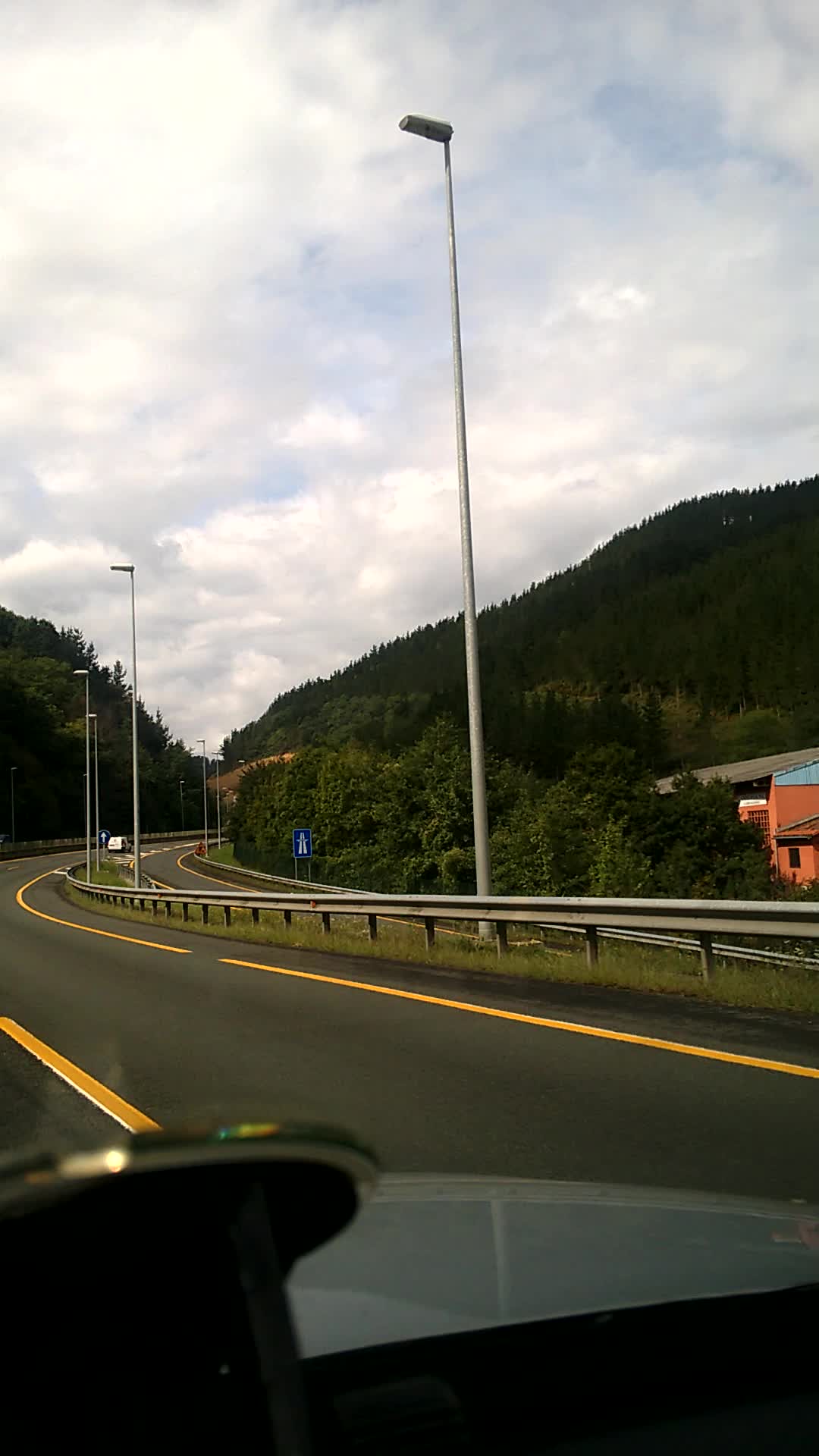This photograph captures a scenic two-lane highway curving off into the distance, taken from the dashboard of a moving car. The road is freshly paved, showcasing vibrant yellow-orange lane markings and bordered by silver metal guardrails. To the right, a large, tree-covered rock structure, possibly a mountain or hill, dominates the scene with a mix of standard and pine trees. Nestled among the greenery is a small, neon orange building with a blue roof, potentially a house or storefront. Several tall, silver light poles line the road, their rectangular tops unlit under the blue sky peppered with white clouds. In the distance, a blue road sign is visible, though its symbols are indiscernible. The vehicle's dark gray exterior is slightly visible, with the black dashboard and a device mounted on the windshield partially in the frame. The road ahead hints at a merging lane, and rolling green hills add to the landscape's natural beauty, creating a serene yet dynamic composition.